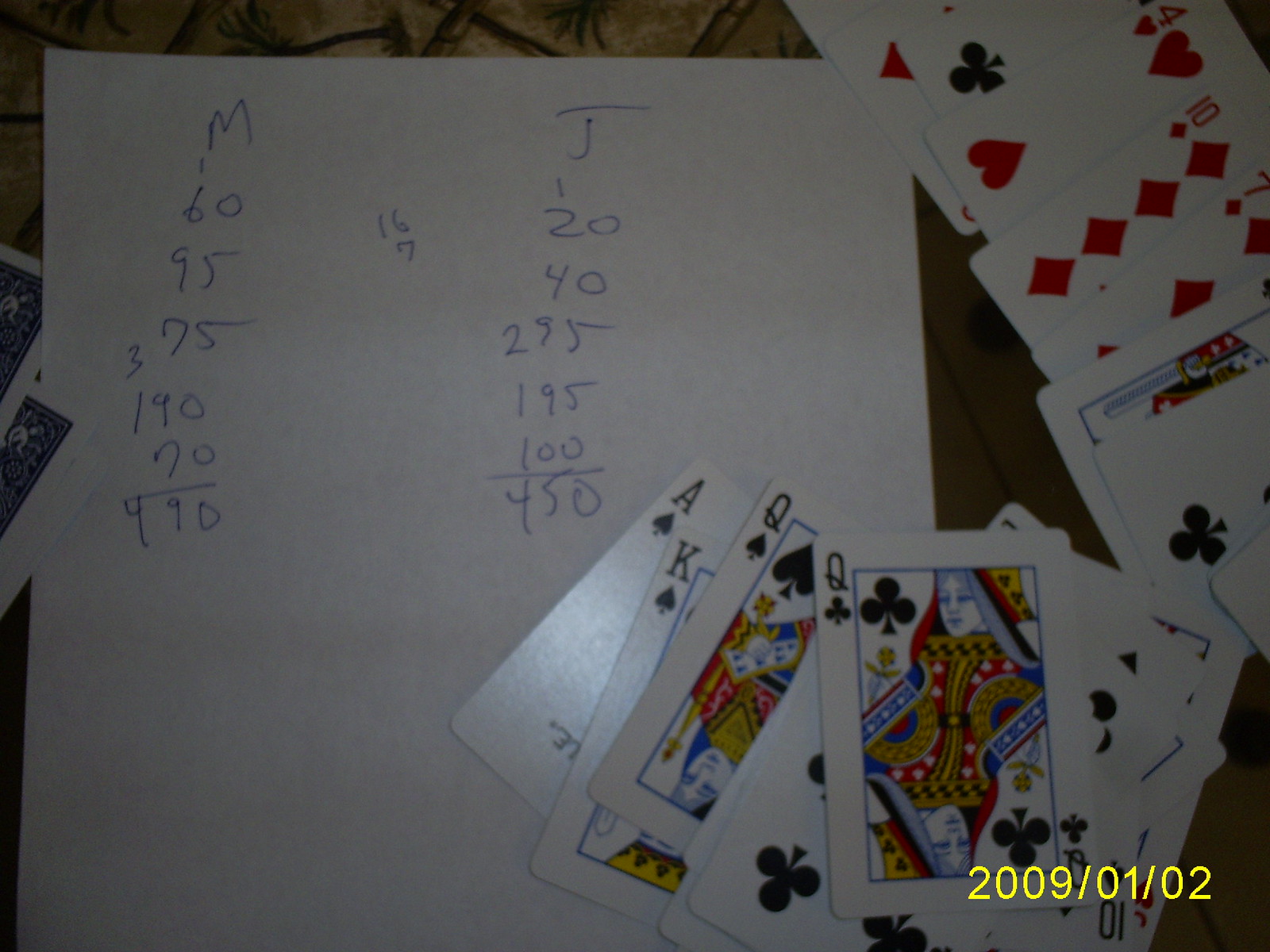A cluttered arrangement of playing cards lies sprawled across a table with a piece of paper partially nestled beneath them. The Ace of Spades, King of Spades, Queen of Spades, Queen of Clubs, Ten of Diamonds, and Seven of Diamonds are prominently displayed among the scattered cards. Below them, the paper appears to be a score sheet, featuring two columns labeled "M" and "J". The scores for "M" are meticulously listed as 60, 95, and 375, summing to a total of 490 points, while "J" enumerates a total of 450 points. Additional writing between the columns includes the numbers 16 and 7, possibly results of quick mental calculations. In the bottom right corner of the paper, a date is clearly noted: February 2, 2009, marking the day of the game. The scene suggests the aftermath of a five-round card game, though the specific game remains unidentified.